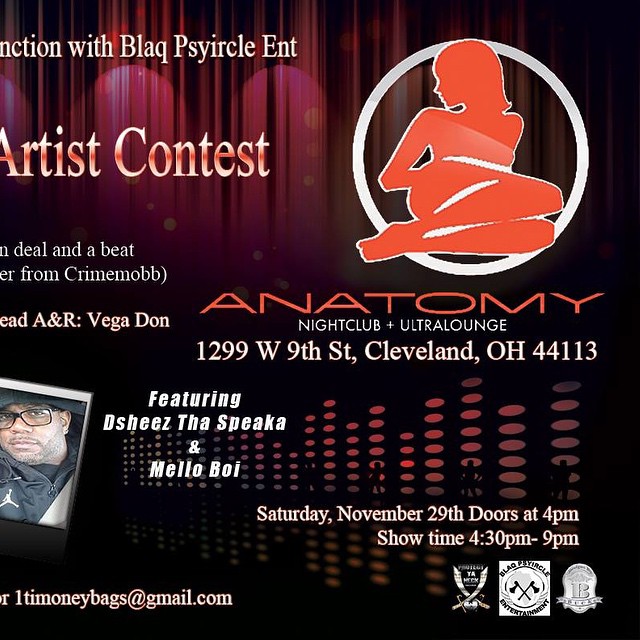The image is an advertisement for the Anatomy Nightclub and Ultra Lounge, located at 1299 West 9th Street, Cleveland, Ohio 44113. The background of the ad is primarily black with red accents, resembling a red curtain at the top. The center of the poster features the word "Anatomy" in bold, red uppercase letters. In the upper right corner, there is a white circle containing the silhouette of a woman sitting with her knees bent, styled in red but outlined in white. 

The advertisement promotes an Artist Contest with the opportunity to secure a deal and a beat from Crime Mob, with Head A&R Vega Dawn. There's a detailed close-up of a black gentleman wearing a black Jordan jacket, a hat, and black-framed glasses. Next to his picture, it announces "featuring Dejeej the Speaka and Mellow Boy." 

The event is scheduled for Saturday, November 29th, with doors opening at 4 p.m. and the showtime running from 4:30 p.m. to 9 p.m. At the bottom right, the ad includes three unidentified logos and the contact email "onetime moneybags at gmail.com" (1timoneybags@gmail.com).